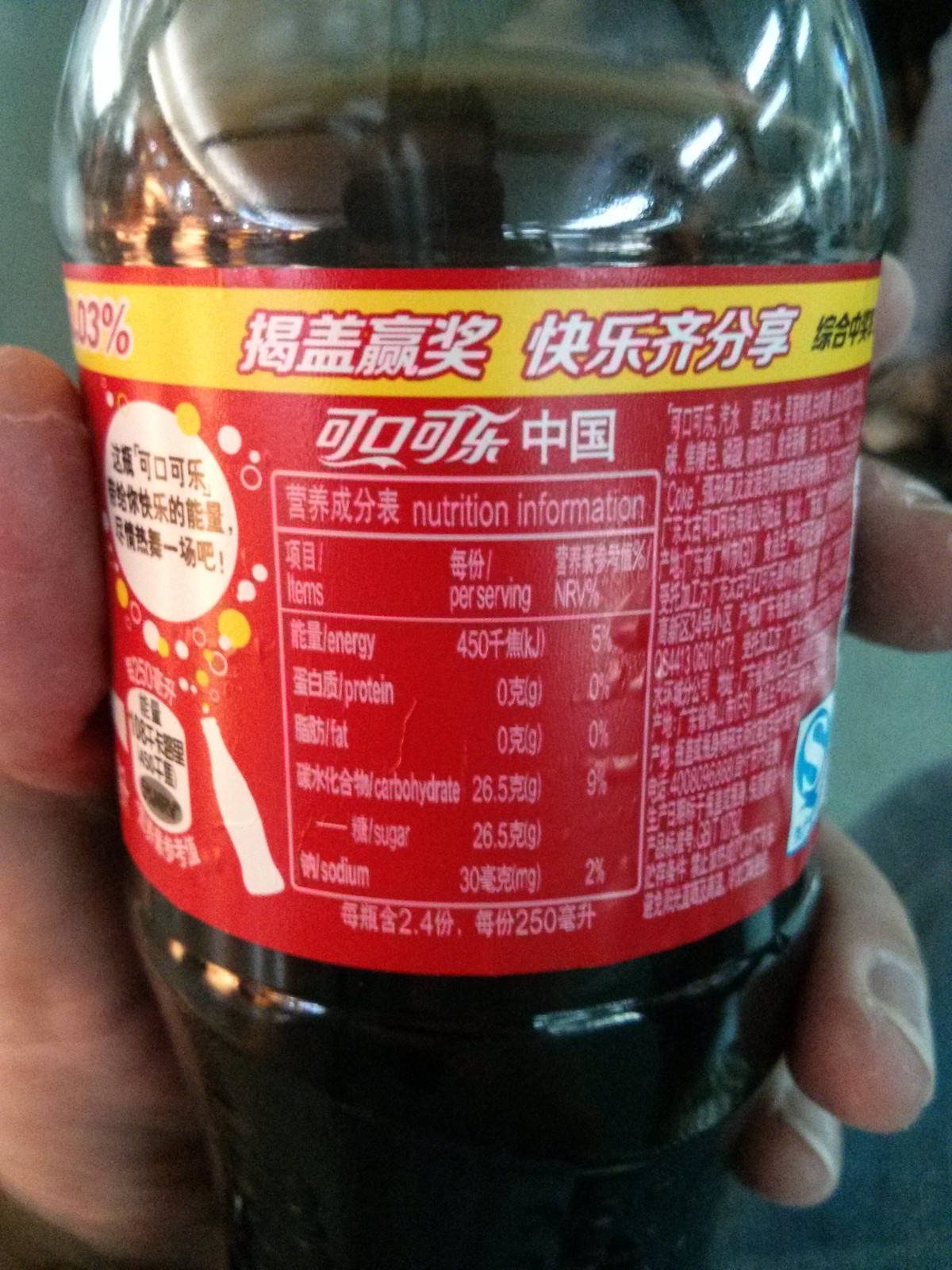A person is holding a plastic bottle of dark-colored cola, likely Coca-Cola, marked by a red label with a yellow border at the top. The individual's thumb, slightly peeling at the tip, grasps the left side of the bottle, while their fingers wrap around the right. The label, adorned with a white text, predominantly features Chinese writing. The nutrition panel, also in Chinese, details energy per serving, protein, fat, carbohydrates (noting specifically 26.5 grams of sugar), and 30 milligrams of soda. Reflections of fluorescent light fixtures are visible on both sides of the bottle, and at the bottle’s top is the person’s partial reflection with their forehead, hair, and the front of their phone obscuring their face. Centered within the label is an image of a traditional glass soda bottle with a long neck and tightened waist, reinforcing the identification of the beverage as Coca-Cola.